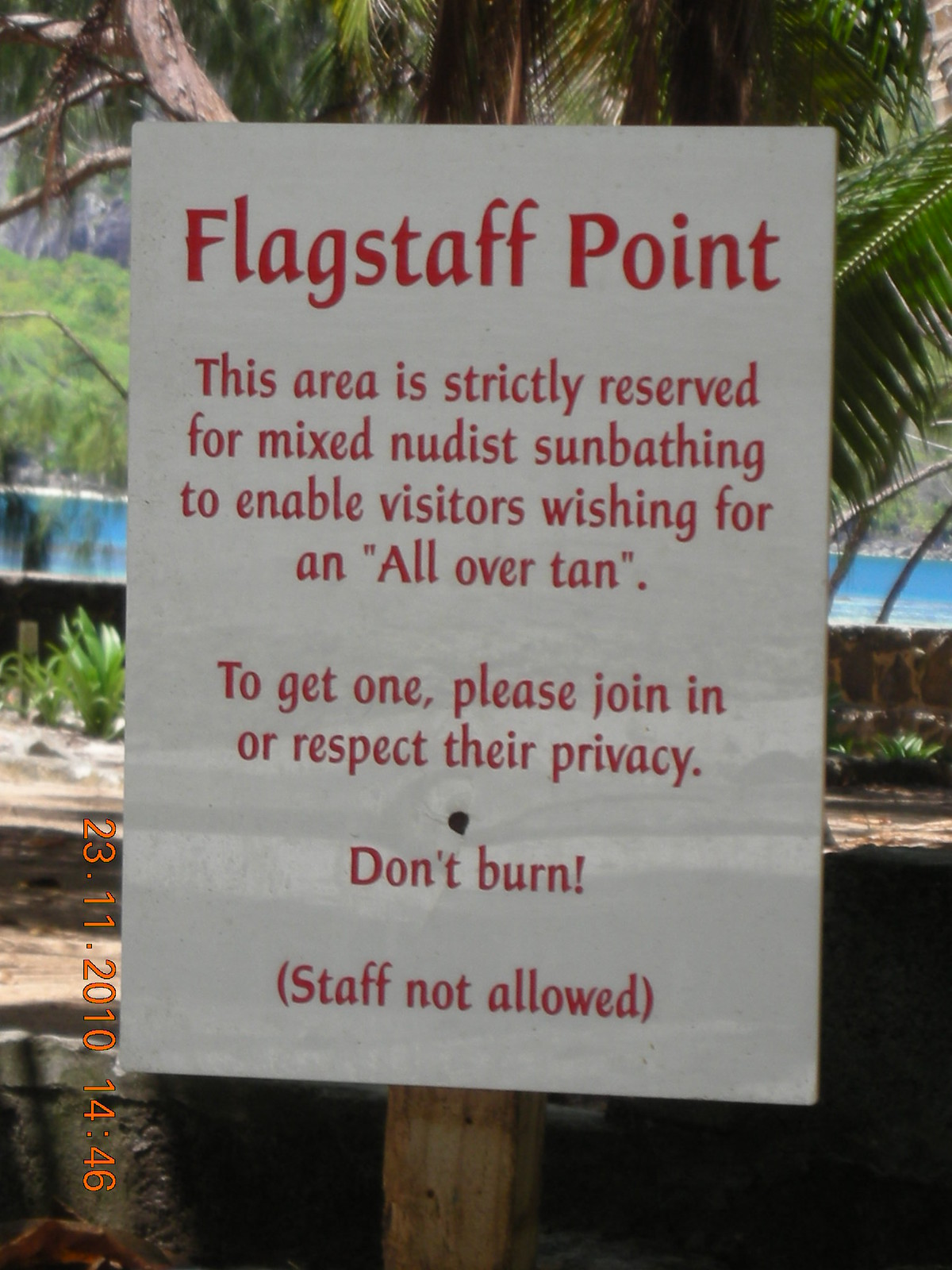This outdoor daytime photograph, taken in portrait mode, showcases a rectangular white sign mounted on a wooden post. The sign features bold red text at the top that reads "Flagstaff Point." Beneath this, in smaller red text, it states, "This area is strictly reserved for mixed nudist sunbathing to enable visitors wishing for an all-over tan. To get one, please join in or respect their privacy. Don't burn!" It also notes in parentheses, "(staff not allowed)." On the lower left corner of the sign, typed vertically in orange, is the timestamp "23.11.2010 14:46." The background includes a picturesque scene with a palm tree, crystal blue water, and various greenery such as plants and shrubs. A small stone retaining wall is visible at the base, giving way to a sandy surface surrounded by lush vegetation.